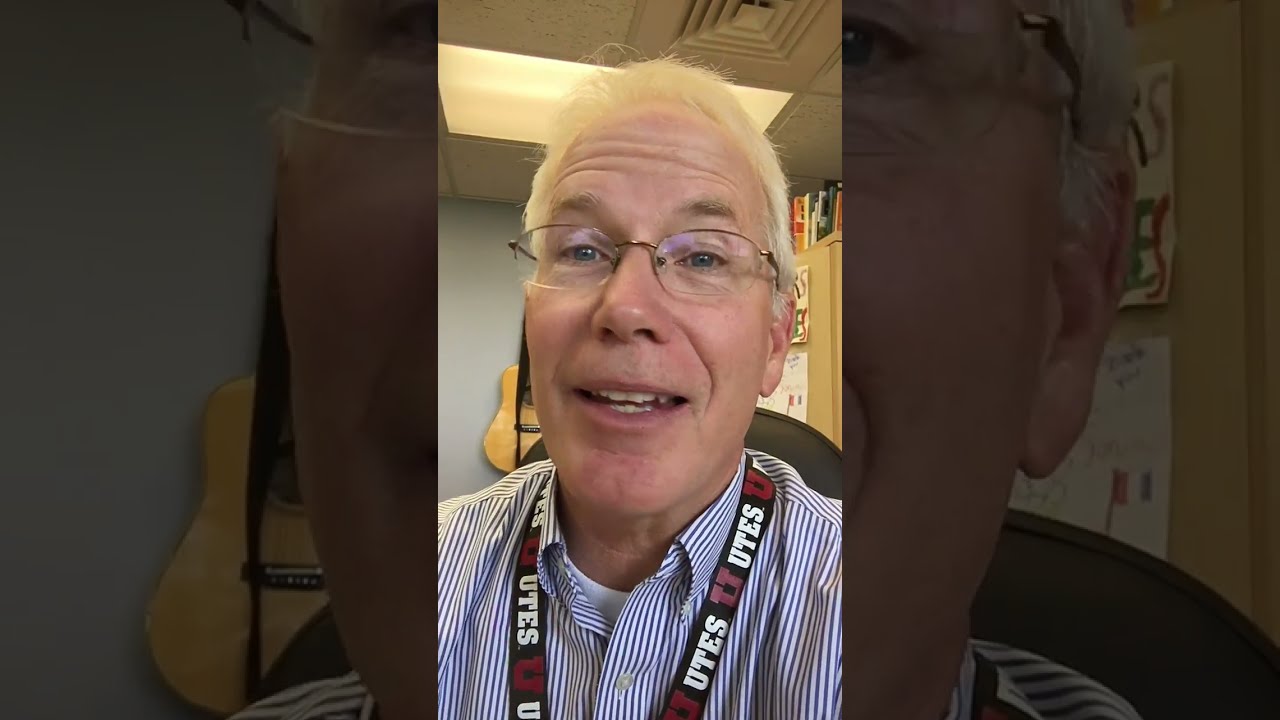This close-up image captures an older Caucasian man, seated and smiling cheerfully with his mouth open, revealing both sets of teeth. He has thin, metal-framed glasses and blue eyes, and his hair is predominantly gray with white strands. He wears a well-ironed blue and white striped dress shirt over a white undershirt, the collar of which is slightly visible. Around his neck hangs a lanyard emblazoned with a red 'U' and the word 'Utes' in white text, accompanied by a trademark symbol, indicating his affiliation with the Utah Utes, possibly hinting at a role in an academic or youth-related position.

In the background, a partial view of an acoustic guitar is visible hanging on the light gray wall to his left. To the right, there is a shelf filled with books and a cupboard adorned with hand-drawn posters, suggesting an academic or office setting. The room is brightly lit, casting a positive and lively atmosphere that complements the man's happy demeanor, further emphasizing his apparent enjoyment of life and his educated, professional persona.